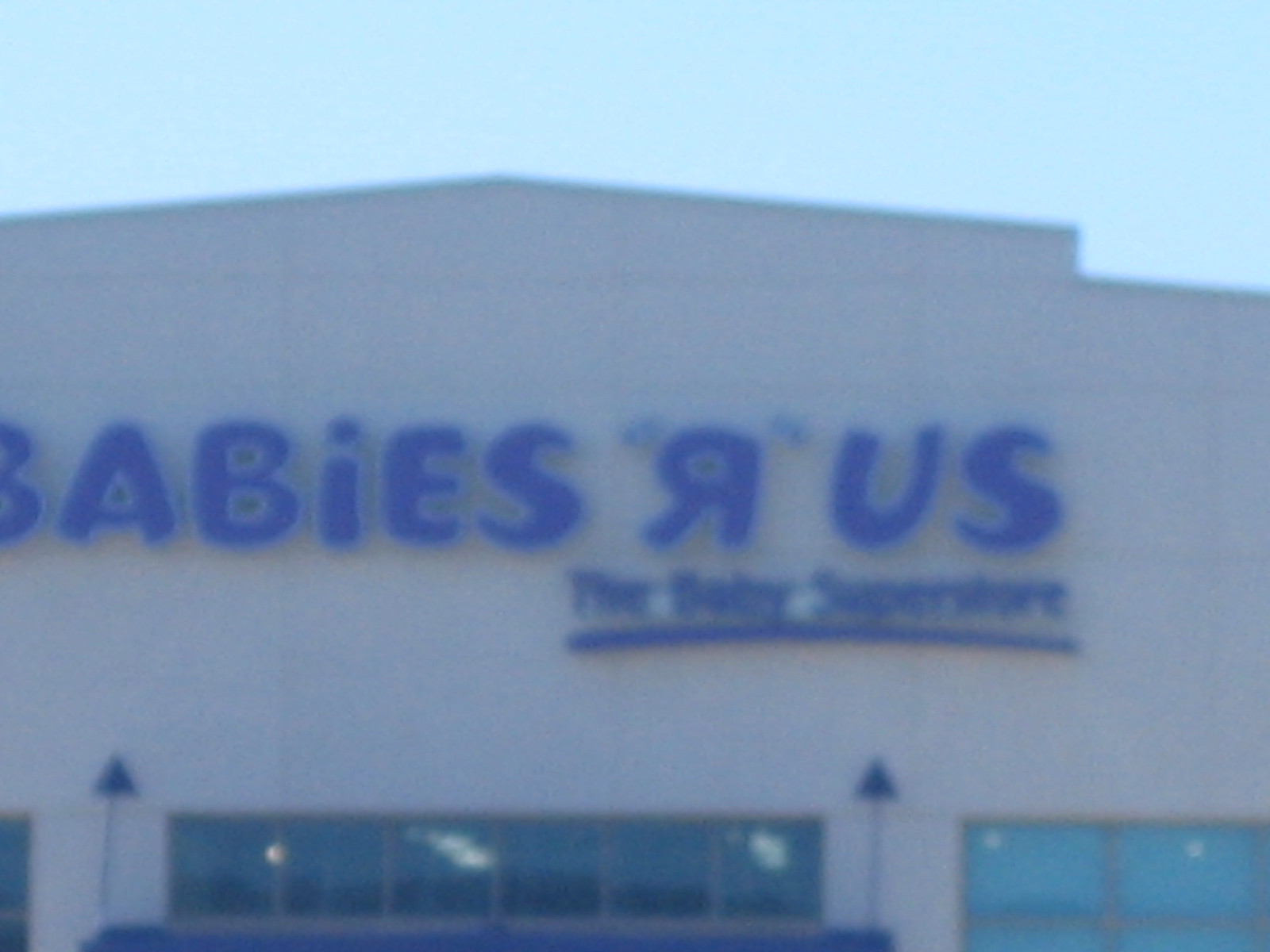This daytime photograph shows the exterior of a large Baby's R Us store, somewhat out of focus and grainy. The building stretches fully across the image, featuring a light tan facade. Prominently displayed at the top in deep blue letters is the store's name, "Baby's R Us," with the signature backward "R" enclosed in quotation marks. Below this main sign, in smaller text, are the words "The Baby Superstore," underlined for emphasis. The building's front is lined with shiny glass doors and multiple sections of windows, the most notable being a set of three windows in the center, flanked by two blue arrows pointing upwards. The sky at the top of the image is a clear, light blue with no clouds in sight. The building itself has a slightly angled roof, adding to its tall, warehouse-like appearance. Despite the blurred quality of the photo, one can discern fluorescent lights inside the store, running down the aisles.